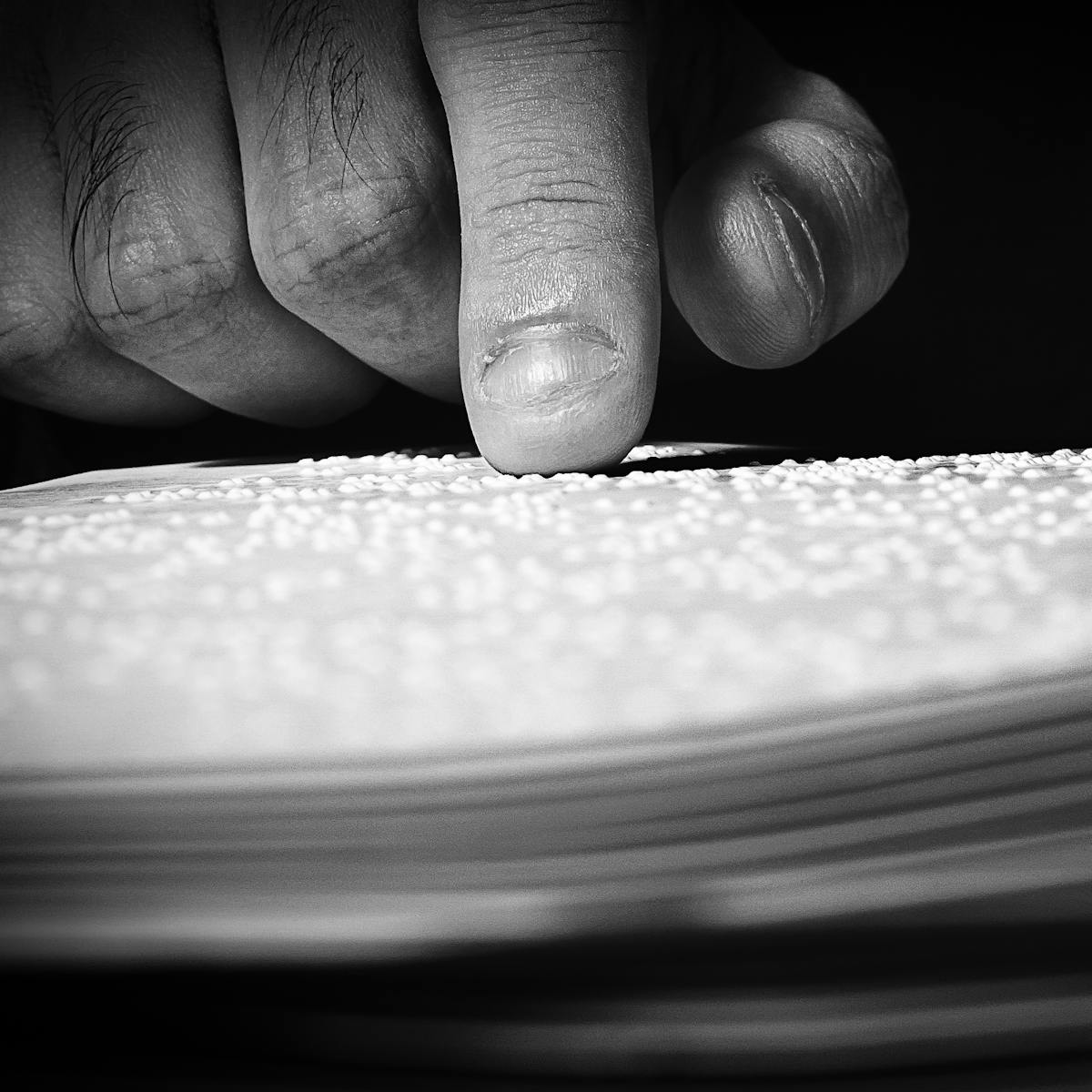The black-and-white photograph features a close-up, zoomed-in view of a male hand, identifiable by the visible dark hairs on the third and fourth fingers. The hand's palm faces downward, with the pointer finger actively pressing down on an object. Only the fingers are shown, with short fingernails, set against a black background. The fingers are touching what appears to be an open book with white, grainy dots across its surface, resembling Braille text. This textured material covers the lower to middle third of the image and suggests layers, hinting at the multiple pages of a Braille book. The overall scene evokes a moment of tactile reading, characterized by its intricate detail and contrast.